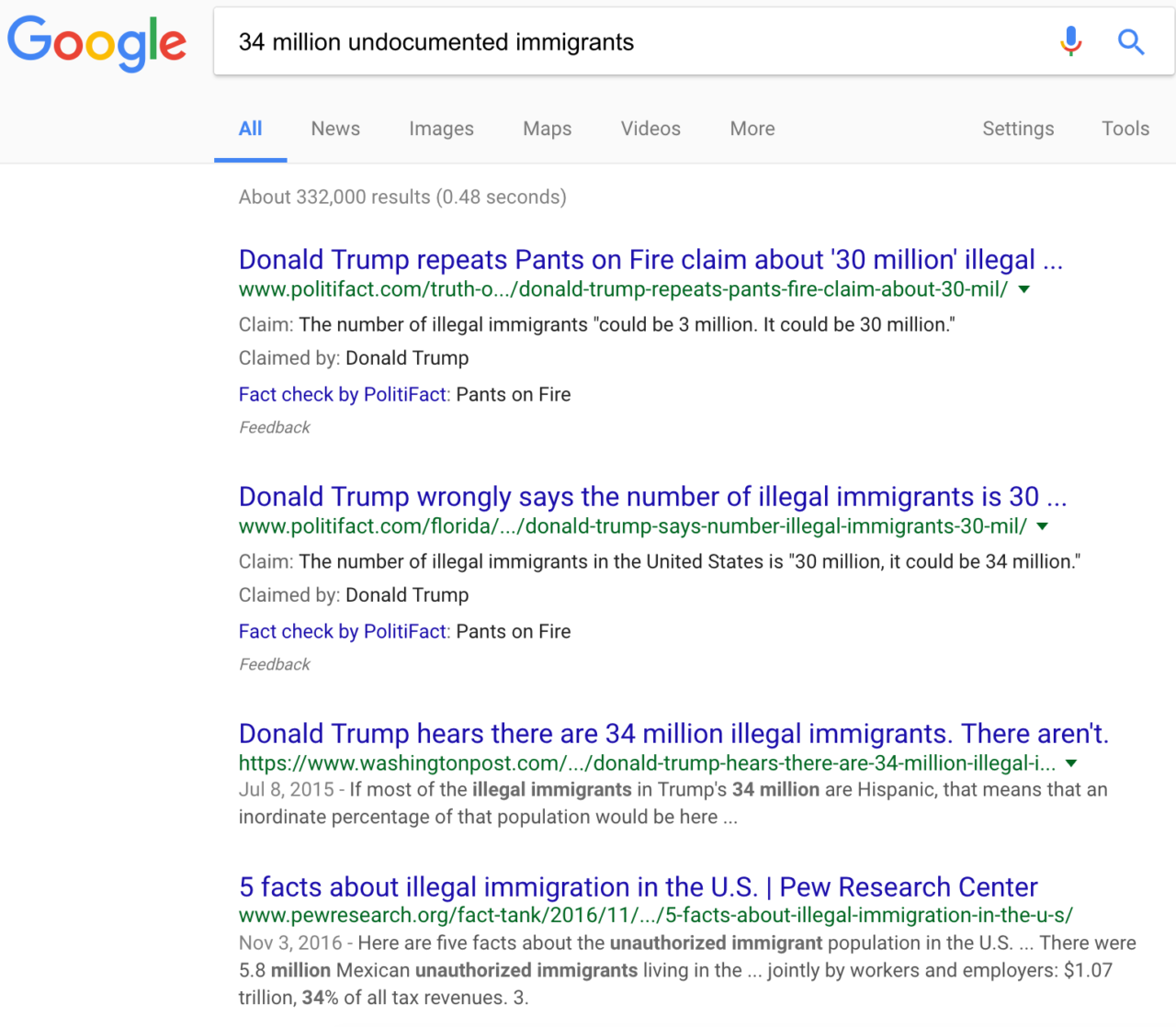The top left corner displays the Google logo. A search query reads "34 million undocumented immigrants." The search results interface includes familiar elements: a microphone icon, magnifying glass icon, and tabs labeled "All," "News," "Images," "Maps," "Videos," and "More." It also shows "Settings" and "Tools."

The search returns about 332,000 results, processed in 0.48 seconds. The first visible result is an article headline stating, "Donald Trump repeats pants on fire claim about 30 million illegal immigrants." The snippet below discusses that the number of undocumented immigrants could be 3 million or as high as 30 million, as claimed by Donald Trump. It also mentions Politifact's "Pants on Fire" rating for Trump’s claim. A URL is cited: www.politifact.com/florida/...

Additional text in the search result snippet reiterates that Donald Trump has claimed there are 30 million illegal immigrants in the United States. Another snippet suggests he might have asserted even higher numbers, such as 34 million. It is mentioned that Trump’s exaggerated figures are fact-checked and debunked by Politifact. The feedback loop suggests Trump’s 34 million figure is incorrect, noting that most undocumented immigrants he refers to are Hispanic.

A linked article from the Pew Research Center presents "Five facts about illegal immigration in the U.S." It highlights that there are approximately 5.8 million Mexican unauthorized immigrants in the U.S., contributing over $1.07 trillion in revenue from their combined work efforts.